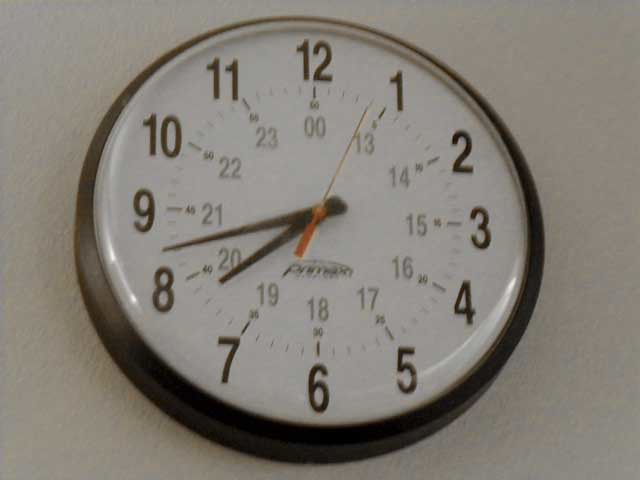This striking close-up image features a Primax clock against a pristine white background. The clock boasts a sleek black border that frames a white face adorned with bold black numbers. Interestingly, the clock is equipped with dual time markings, offering both standard and military time; for instance, the number 1 is accompanied by a smaller 13. A vivid red second hand adds a pop of color, while the primary black hour and minute hands point to 7:43, aligning with either 7:43 a.m. or 19:43 (7:43 p.m.), depending on the context. This detailed shot emphasizes the clock's functionality and aesthetic appeal.